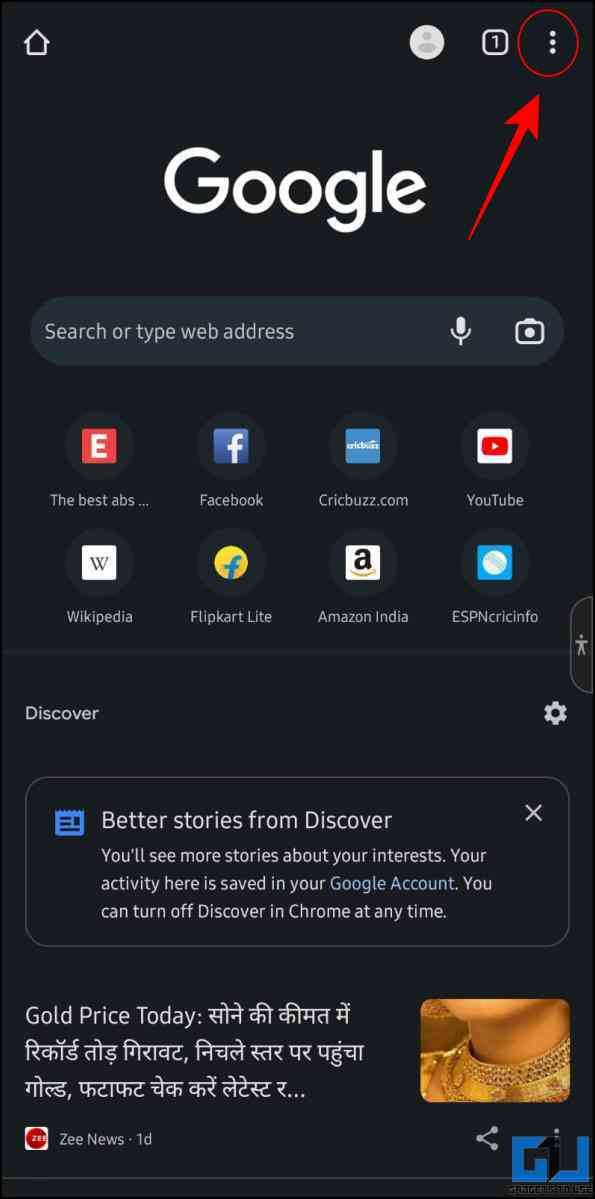This image displays a vertically-oriented rectangular webpage with a black background. In the top left corner, there is a small gray house icon. To its right sits a gray circle featuring a darker gray silhouette of a person. Next, there is a gray square containing the numeral "1," followed by three vertical gray dots on the extreme right.

Below this top section, the webpage prominently displays the word "Google" in white text. An arrow directs attention to the three dots mentioned earlier. Underneath the "Google" text is a search bar.

Moving further down the page, there are various icons representing different suggestions. Starting from the left, the first suggestion is an "E" in white within a red box. To its right is the Facebook app icon depicting a white "f" on a blue background. Continuing to the right, there's a blue square with white writing that is illegible due to its small size. The furthest icon on the right in this row is the YouTube app icon, characterized by a red square with a white play button.

In the next row of suggestions starting again from the left, there is a white box with a "W" symbolizing Wikipedia. Beneath this icon, the text reads "Wikipedia." Moving to the right, there is a yellow circle featuring a blue "F," the associated text under it is unreadable. Continuing rightward, a white box houses an "A" symbolizing the Amazon app, with the text "Amazon India" beneath it. The final icon on the furthest right is a blue box with a white circle inside bearing the text "ESPNCRICINFO."